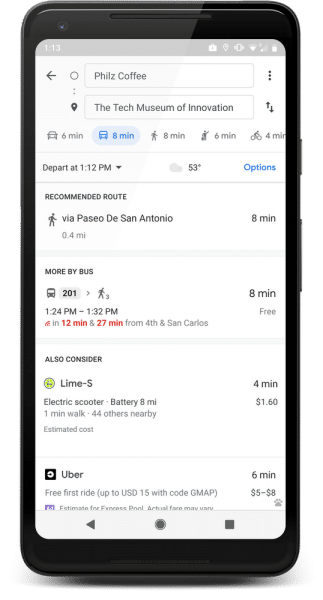The image displays the results of a direction search on a black smartphone. At the top of the screen, a light purple banner shows the time, "1:13 PM," in white text on the left side. On the right, several icons are visible, including a battery icon indicating a charge level of approximately 60-70%.

Beneath the banner, on a white background, two boxes are displayed. The top box contains the original destination, "Philz Coffee" (spelled P-H-I-L-Z Coffee), in gray text. The bottom box indicates the new destination, which is the "Tech Museum of Innovation."

Below these boxes, the screen shows navigation details. It indicates that the user is traveling by car and highlights an eight-minute route in blue. This section notes a departure time of "1:12 PM" and the current temperature of "53°F." On the far right, there is a bright blue button labeled "Options."

Further down, it specifies the "Recommended route" in gray text and includes an icon of a person walking. It also mentions the pathway, "Via Paseo de San Antonio," in gray text.